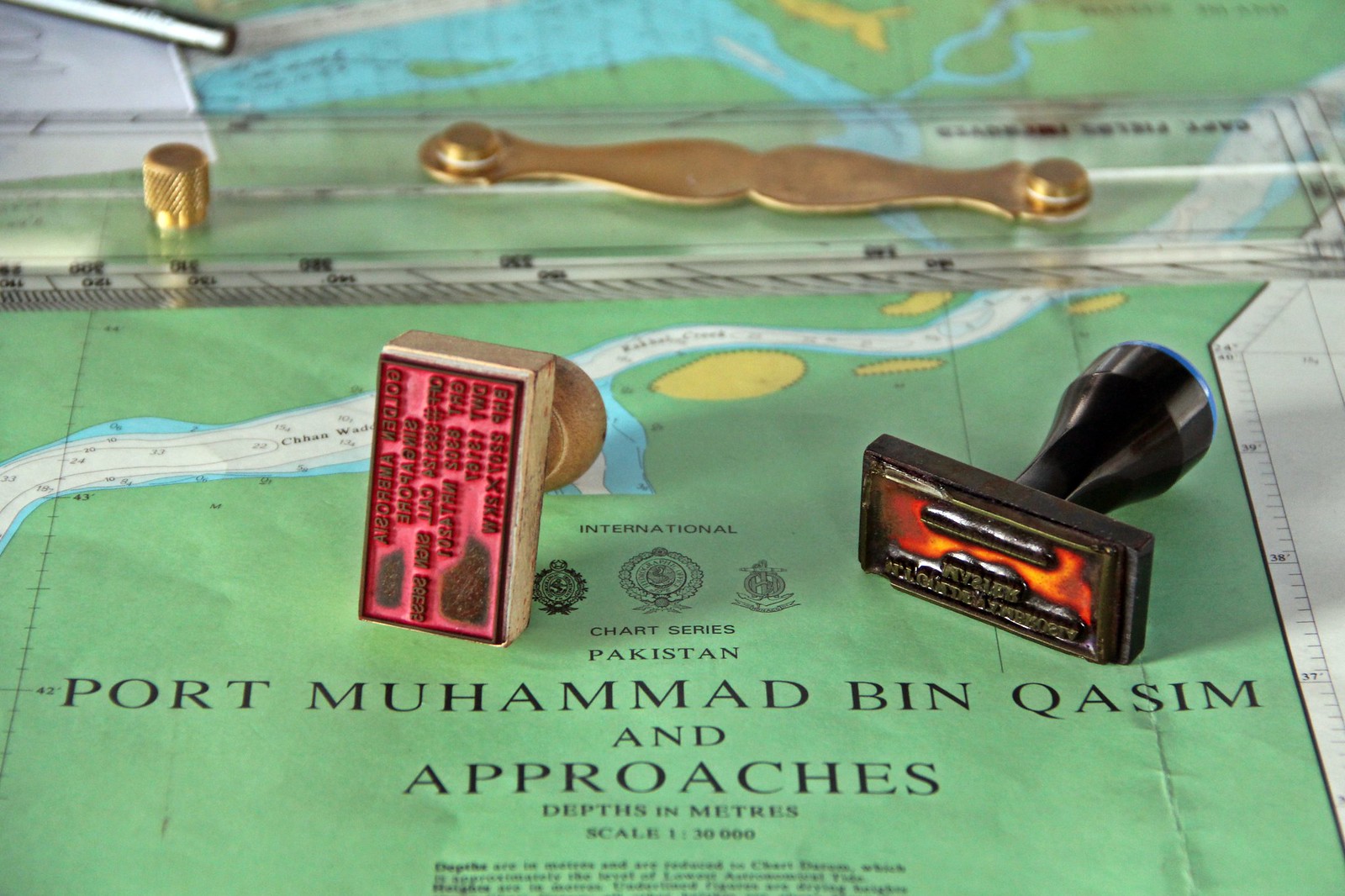The image depicts a partial nautical map, intricately detailed with various textual and graphical elements. The map, set against a green background, prominently displays in black letters, "Port Mohammed Bin Qasim," and “Approaches,” along with the words "Depths in Meters" and other smaller, less readable text. On the right-hand side of the map, there appears to be a ruler or similar measuring tool in white and black. At the top, a brass metal piece with a removable knob possibly serves as a protective covering or measuring device for the map. Two rubber stamps rest on the map: one on the left is a conventional beige-handled stamp with a pink rubber base, and the other on the right features a black handle with a black and red rubber base. Additional colors such as white, blue, and orange adorn the map, providing further navigational details and measurements.